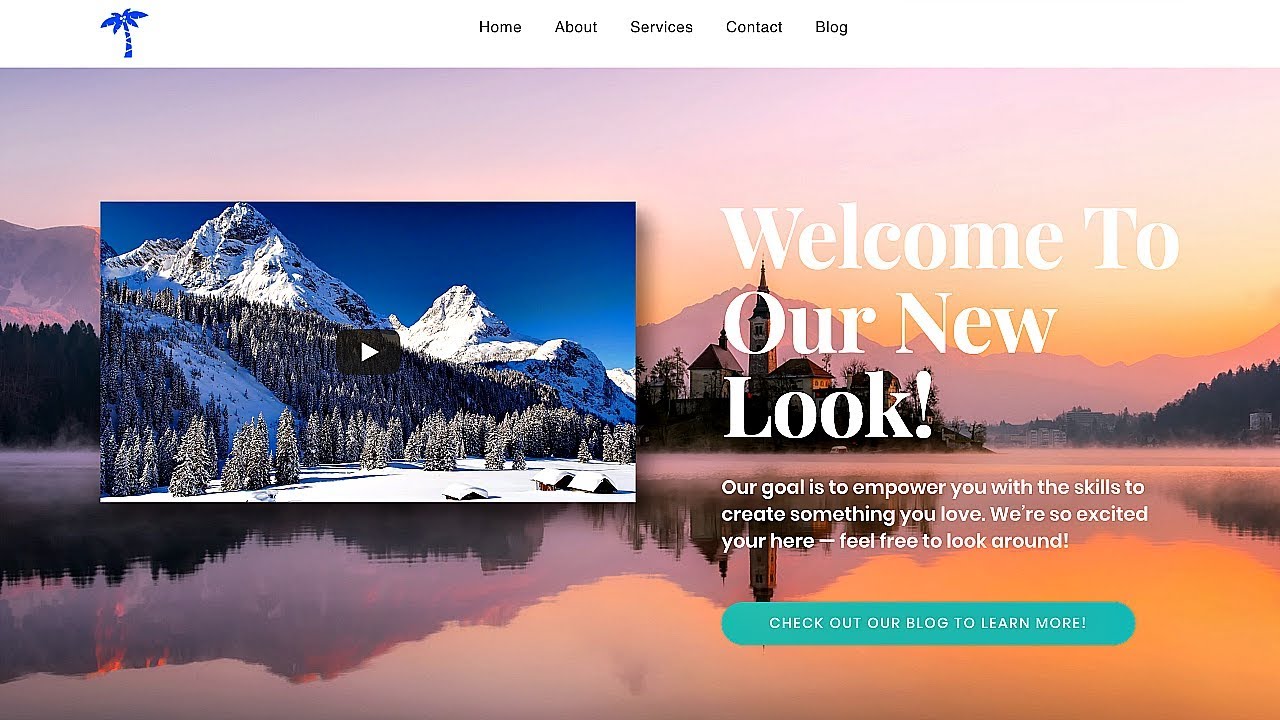This web page exemplifies a modern, revamped design with a variety of content elements aimed at enhancing user engagement. At the center of the page, there's a paused video featuring a serene landscape of snowy mountains and a forest, aptly captioned "Welcome to Our New Look." The text beneath emphasizes the organization's mission to empower users with skills to create something they love, expressing excitement about the visitor's presence. Notably, there is a minor typo: "your" should be "you're," which slightly detracts from the professional presentation.

Navigation links are conveniently located at the top of the page, including Home, About, Services, Contact, and Blog, making it easy for visitors to explore different sections. A palm tree image in the top-left corner appears to represent the company's logo, although there is no visible text indicating the company name, which might be a point of confusion for some users.

Additionally, the webpage encourages visitors to explore further by inviting them to check out the blog for more information. Overall, the new design is clean, modern, and user-friendly, representing a significant improvement over the previous version, even though the older page is not depicted for comparison. Despite the minor typo, it stands as a commendable start to their revamped online presence.